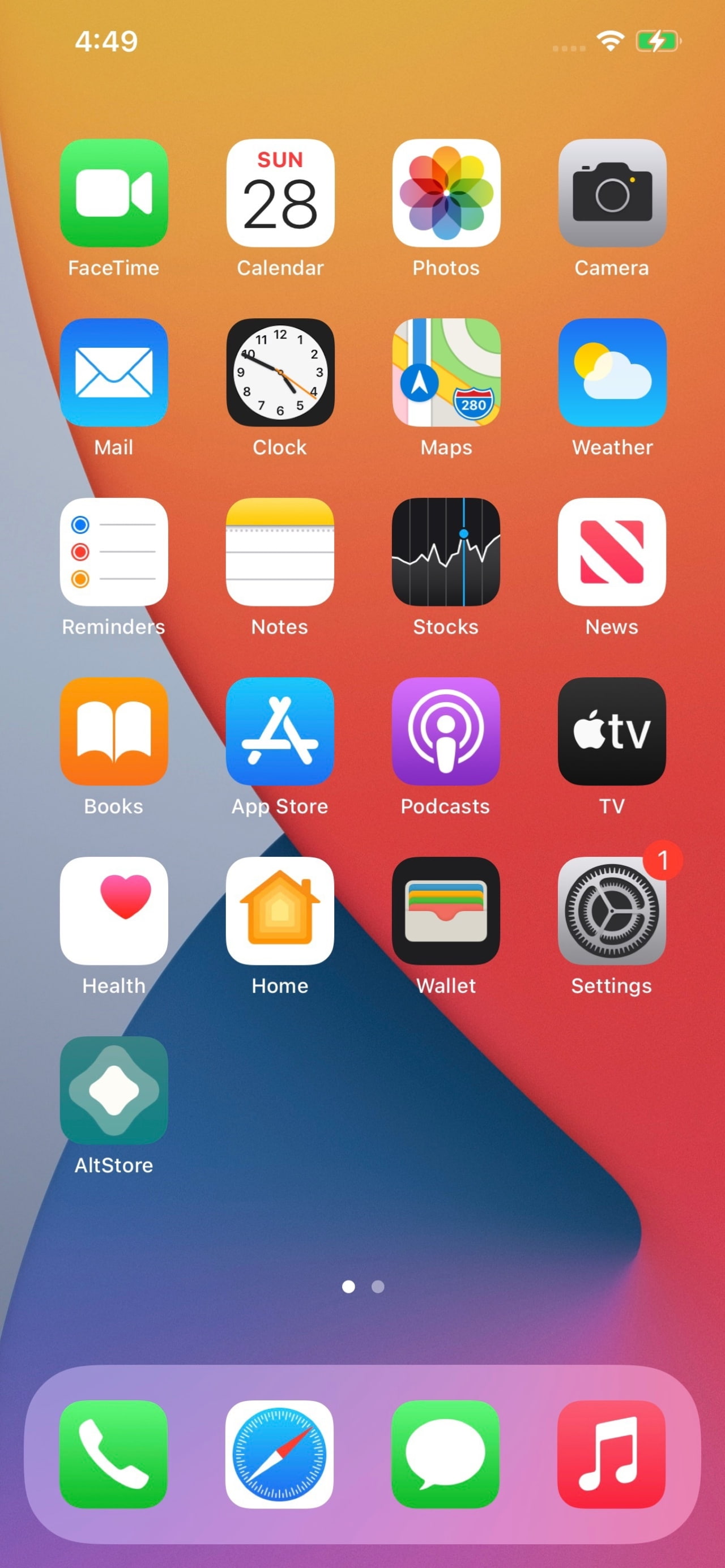This screenshot captures the home page of an iPhone running on the iOS platform. The background is a striking mosaic of red, blue, and gray shapes. The home screen exhibits a structured array of application icons, organized into six rows—five rows containing four icons each, and a single additional icon situated at the bottom left.

Prominently displayed at the screen's bottom center, within a light gray dock, are four frequently used application icons: the Phone app, Safari browser, Messages app, and Music app. These apps are easily accessible for convenience.

At the top of the screen, the current time is shown as 4:49 PM in the top left corner. In the top right corner, there are indicators for the data and wireless signal strength, alongside a fully charged battery icon featuring a lightning bolt, indicating the phone is charging.

The various multicolored icons across the home screen represent different apps installed on the device, including FaceTime, News, App Store, TV, and Settings. Notably, the Settings app is marked by a gray icon with black gears and a small red circle with a white number "1" in the top right corner, signifying an unread notification.

Overall, this detailed snapshot vividly conveys the layout and key features of this iPhone’s home screen.